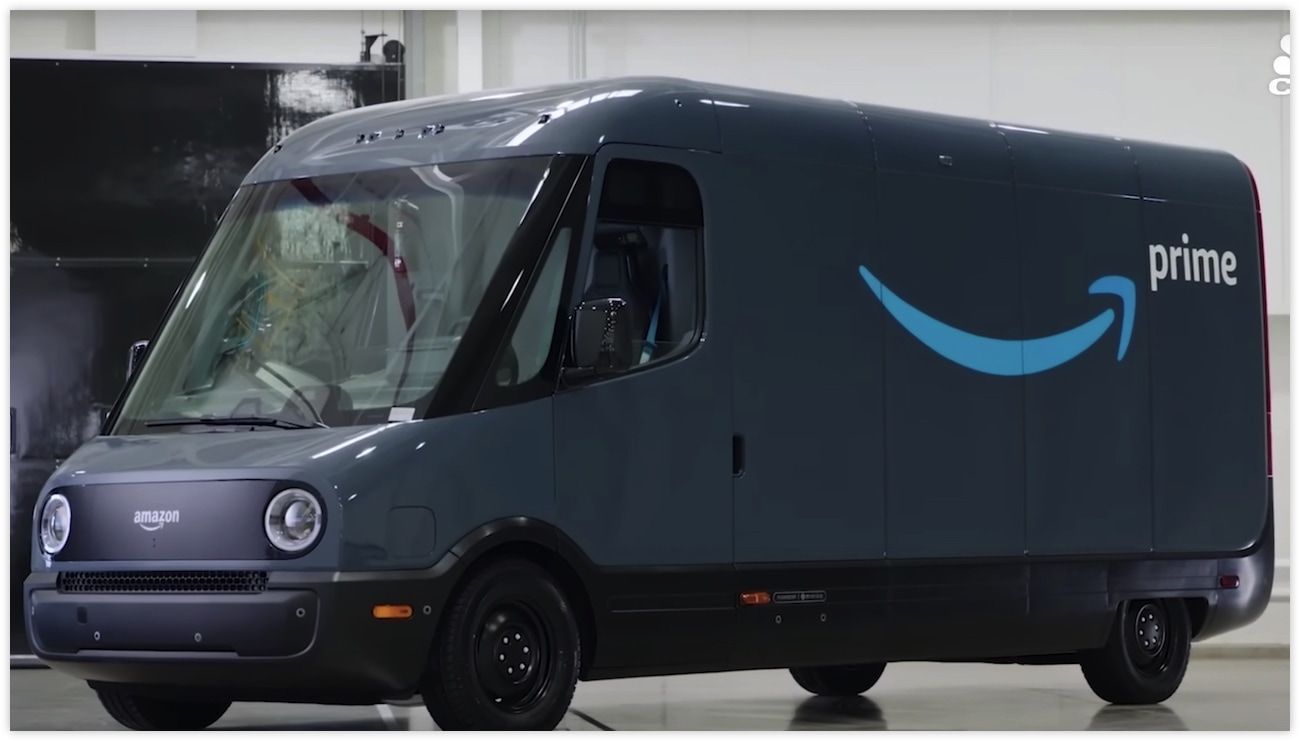This photograph showcases a dark slate gray, near-black Amazon Prime delivery van. On the side, a distinctive blue smile is featured next to the word "prime" in white, indicating its function as a delivery vehicle. The front of the van proudly displays the "Amazon" name with the signature smile logo beneath, both in white, situated between the sleek white headlights. The van itself is designed as a cargo van with rounded edges, eliminating any sharp corners and adhering to a modern aesthetic.

The predominantly dark slate gray color is juxtaposed with purely black elements, such as the tires, accentuating the van's sleek design. The van's exterior is further detailed with two orange hazard reflectors positioned on the sides. The vehicle rests on a polished light gray cement floor that reflects its image, adding to the photograph's overall clarity.

In the background, a large door is visible to the left, set against an unembellished white wall. Inside the van, one can glimpse the driver's black seat equipped with a blue safety belt. The driver’s window is notably expansive, enhancing visibility. This cargo van’s size and structure indicate it is intended for commercial deliveries rather than personal use.